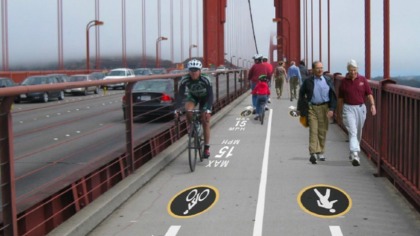The photograph captures a striking image of a large, red bridge bathed in rich, dark copper hues. The bridge features multiple lanes for traffic, with four gray lanes for cars occupying the left side, and a distinct separation between lanes moving in opposite directions. On the right side of the bridge, designated lanes for both bicyclists and pedestrians are visible. The bike lane, marked with a black and white logo and a "max 15" speed limit sign, hosts several cyclists, including one prominent rider wearing a white helmet. Adjacent to the bike lane is the pedestrian lane, identified by a similar black and yellow logo, where a few people, clad in jackets, stroll towards the camera. The rightmost part of the image shows a coppery red fence running parallel to the pedestrian lane. The overall scene is framed against a backdrop of blue skies and punctuated by enormous red pillars and cables supporting the bridge. Streetlights line the left side, contributing to the vibrant atmosphere with colors of black, white, gray, copper, red, green, blue, and brown interspersed throughout the image.